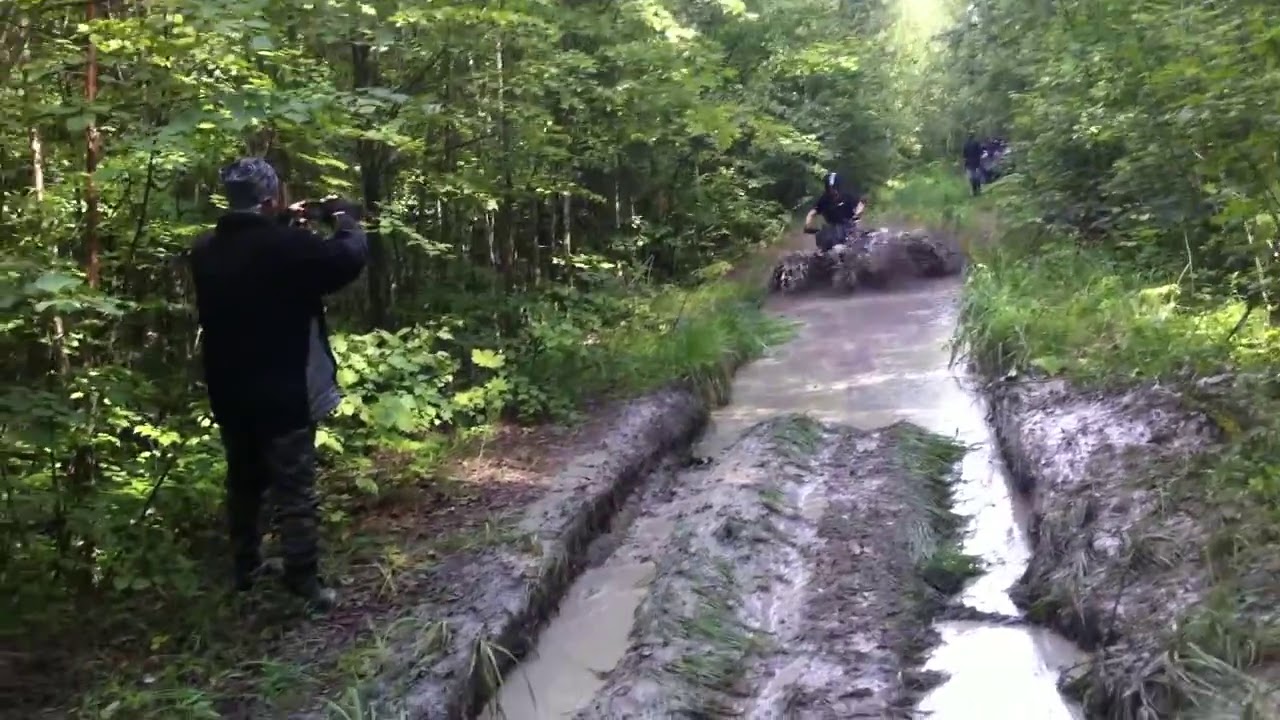In the vibrant depths of a forest, a muddy and heavily rutted dirt road stretches through the greenery. The air is dense with the earthy scent of wet soil and damp leaves, as the surrounding trees are lush with green foliage and dense vegetation. The focal point is a deeply soaked mud trail running through the center of the image, flanked by waterlogged, muddy tracks. 

Near the front and to the left, a person dressed in dark clothing is visibly capturing the action with their phone. Their focus is on the individual at the center, who is navigating a motorbike through this muddy expanse. The motorbike rider appears to be splashing through the water, sending droplets flying amidst the challenging terrain. In the distance, another figure stands slightly pixelated but recognizable, alongside another ATV, hinting at more forthcoming activity. The scene is a dynamic portrayal of mud running in a natural, forested setting, full of energy and the thrill of off-road adventure.